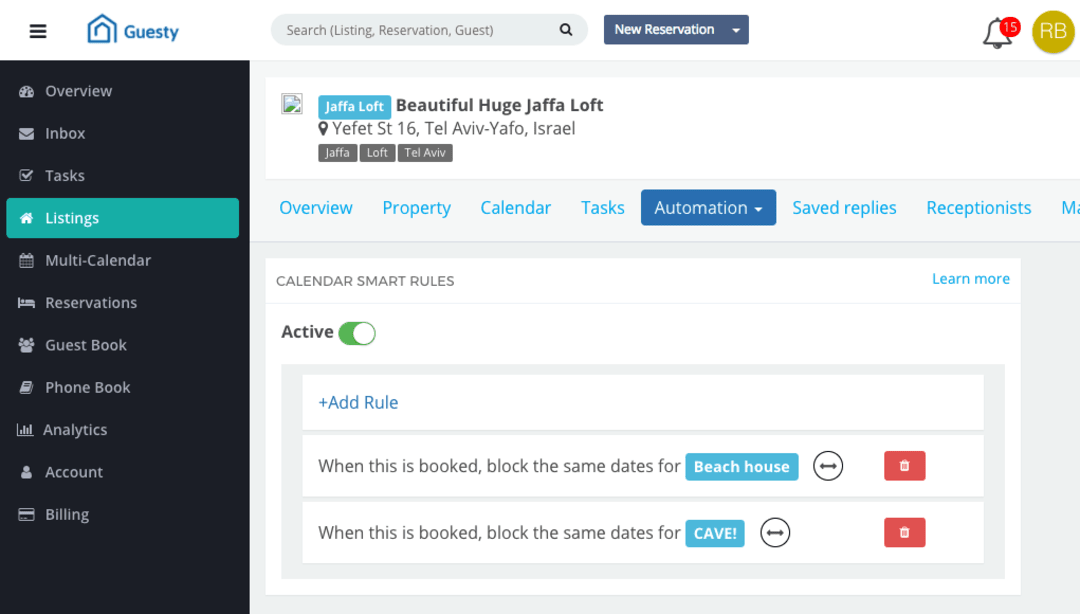The image appears to be a screenshot from a property management website called "Guestry." In the upper left corner, there is the Guestry logo featuring a small house icon next to the site name. A gray search bar labeled "Search listing, reservation, guest" is prominently displayed, accompanied by a blue button labeled "New Reservation" and a bell notification icon on the right side. To the far right, a circular icon containing the letters "R&B" is visible.

The left side of the interface features a vertical black sidebar with various navigation options. One option, "Listings," has been selected. 

The main content area on the right is a gray and white content box displaying a property listing titled "Jaffa Loft - Beautiful Huge Jaffa Loft" located in Tel Aviv-Yaffo, Israel. 

Underneath the description, the "Automation" tab is selected, revealing several settings. One setting is labeled "Calendar Smart Rules," which is currently active, indicated by a green switch. 

Below this, two automation rules are listed:
1. "When this is booked, block the same dates for Beach House," with "Beach House" highlighted in a clickable blue box.
2. "When this is booked, block the same dates for Cave," with "Cave" also highlighted in a clickable blue box.